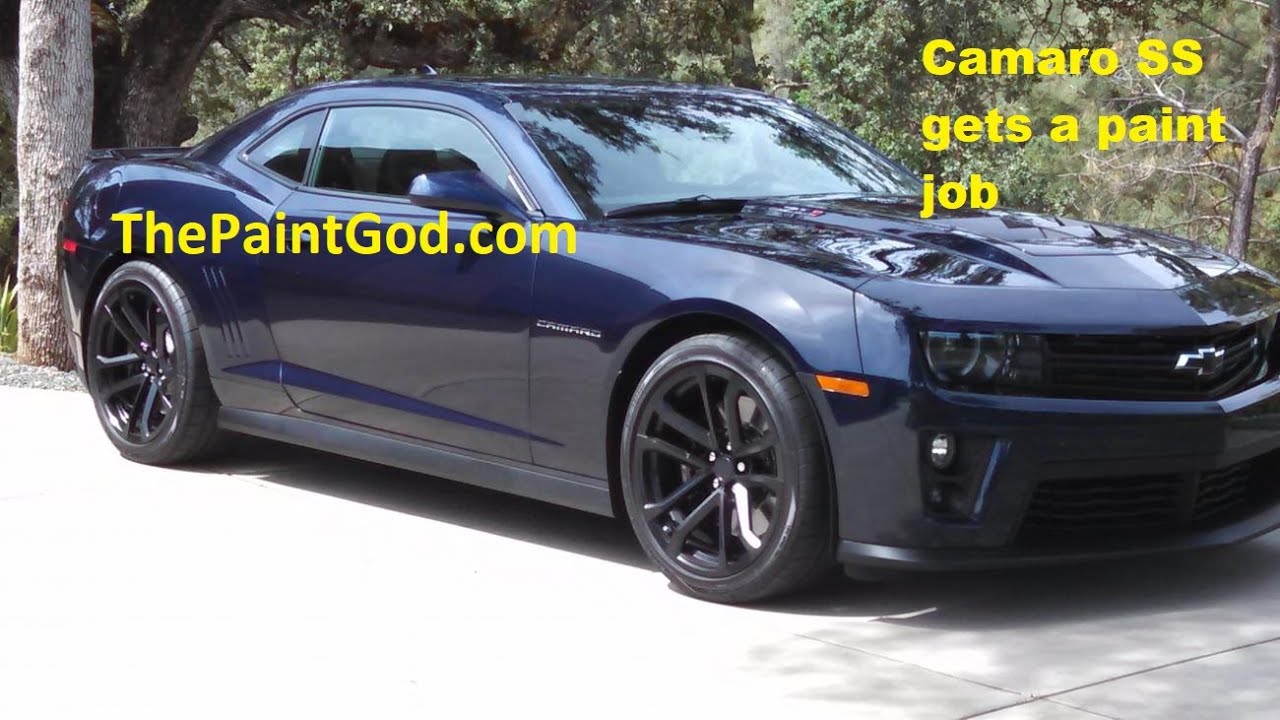This rectangular outdoor photograph captures a freshly painted, glossy dark blue Camaro SS parked on a concrete slab driveway on a sunny day. The sun, shining from the upper left, casts shadows in front of the vehicle, which is angled showing the passenger side. The Camaro, adorned with silver letters spelling its name and a muscle car aesthetic, stands vividly against a lush background of large trees and dense greenery, hinting at a sloping wooded green space. Overlaid on the image in yellow text are two inscriptions: "thepaintgod.com" on the left and "Camaro SS gets a paint job" on the upper right, emphasizing the vehicle's newly minted paint finish.